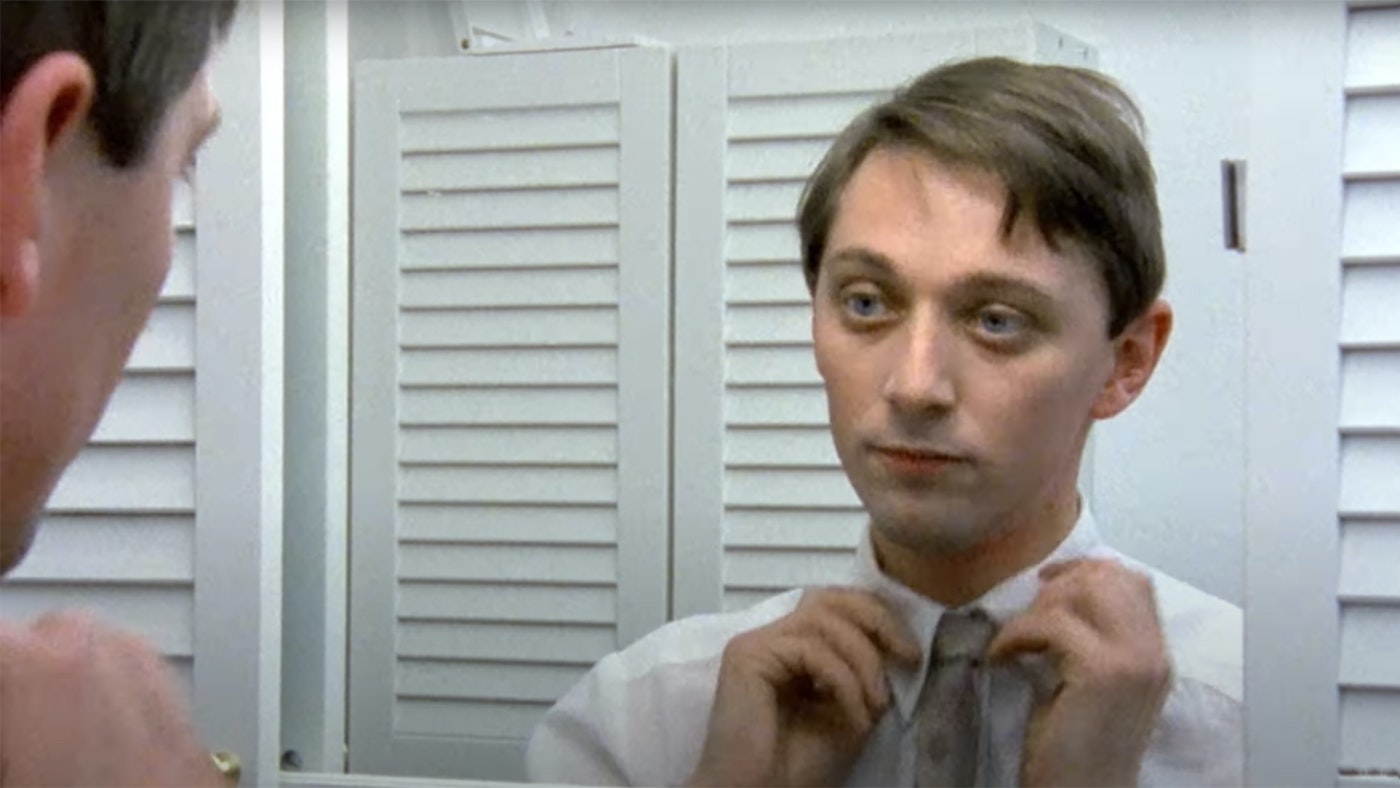The image, likely a scene from a movie, depicts a young, clean-shaven man in his early 20s with light brown hair that is brushed to the side. He has light-colored eyes, possibly blue or blue-gray, and fair skin. The man is standing in a bathroom and is reflected in a mirror as he adjusts the collar of his white, button-down shirt with both hands. He is also wearing a tie, which appears to be in the final stages of adjustment. His expression is blank, with a resting mouth neither smiling nor frowning. The bathroom's white background, including a reflection of a louvered cabinet door and the door to a stall, can be seen behind him. A slight profile of the man is visible on the left side of the photo, but his full face is seen clearly in the mirror, highlighting his focused but somewhat dazed demeanor.